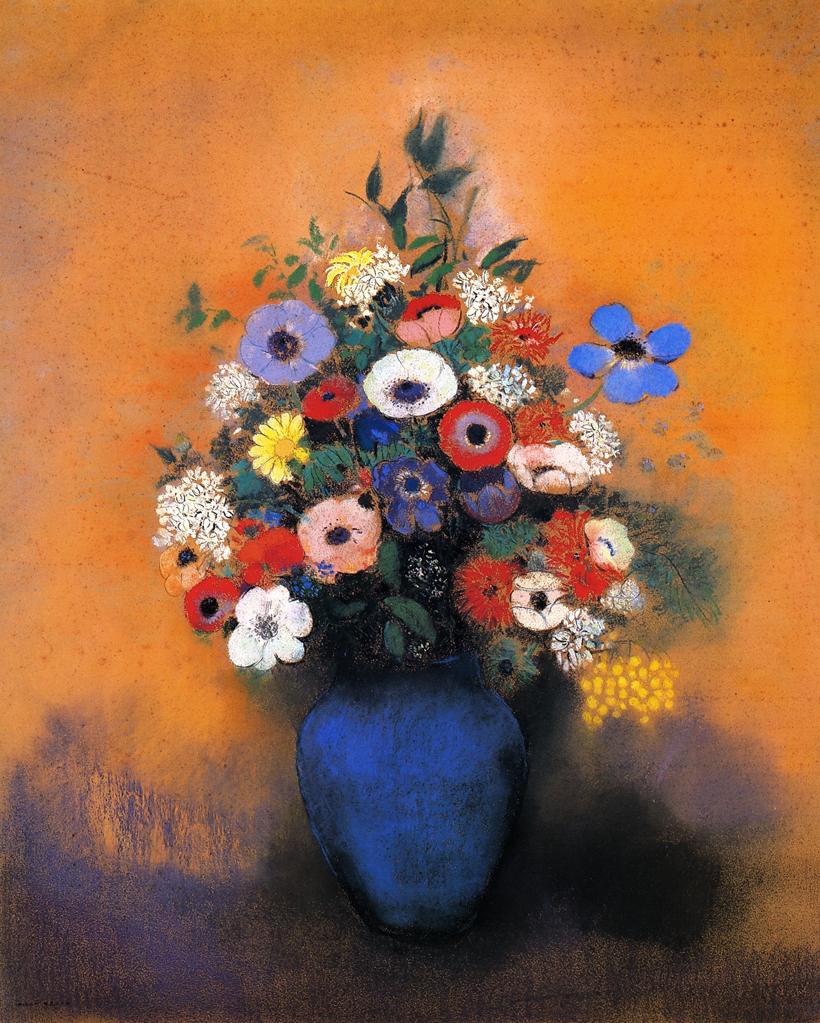This detailed rectangular painting features a striking composition of a vase brimming with an assortment of colorful flowers. Dominating the background is a deep burnt orange hue, speckled with darker orange variations, which covers about 80% of the backdrop from the top downward. Towards the bottom of the painting, the background transitions into a faded area of black and purple, with splatters of blue merging into the darker tones.

Centrally placed at the base of the image is an oval, apple-shaped deep blue vase adorned with black, charcoal-like etchings on its sides. The vase, occupying about a quarter of the painting's height, hosts a diverse bouquet of flowers in various colors and species. The arrangement of flowers forms a diamond-shaped cluster, wider and taller than the vase itself, adding to the visual impact.

The bouquet includes white flowers with round petals, lavender flowers with dark purple centers, and yellow flowers with thin petals. Among them are also blue flowers in shades ranging from pale to dark, red flowers, orange flowers, and some pinkish-purple blooms. The composition is further accentuated by several green leaves interspersed among the flowers.

Overall, this high-definition, text-free artwork combines a rich palette and intricate details, creating a visually captivating scene that celebrates the beauty of a vibrant floral arrangement against an evocative background.